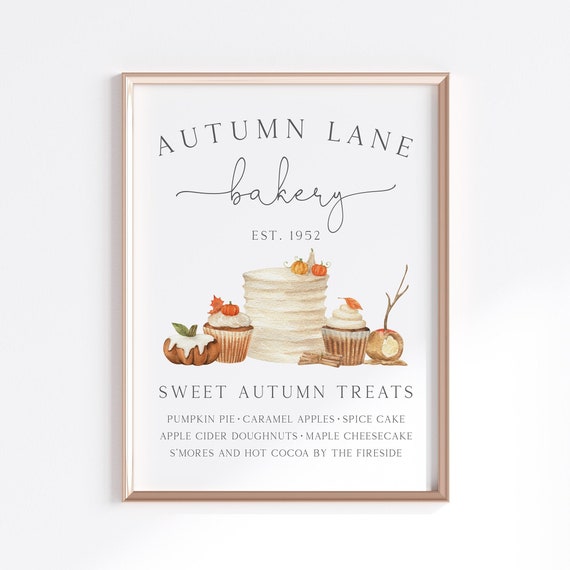This image showcases an elegantly framed sign advertising "Autumn Lane Bakery." The sign features "AUTUMN LANE" in all caps and "bakery" in a cursive script, with "established 1952" written below. Adorned with autumn-themed illustrations, the sign displays fall pastries including an orange frosted pumpkin with a green stem, a cupcake in a wrapper topped with white frosting, an orange pumpkin, and a leaf. Additionally, there is a stack of pancakes topped with small pumpkins, another pumpkin with a leaf, and a partially eaten apple with its stem intact. 

Below these visuals, the text "SWEET AUTUMN TREATS" is prominently displayed in all caps. The menu lists: "Pumpkin Pie, Caramel Apple Spice Cake, Apple Cider Doughnuts, Maple Cheesecake, S'mores, and Hot Cocoa by the Fireside," each separated by bullets. 

The entire print is set against a white background, framed by a thin light copper or gold metal frame, and is hung on a white wall with light shadows. The various fonts used add to the rustic charm, creating a cozy and inviting advertisement for seasonal bakery delights.